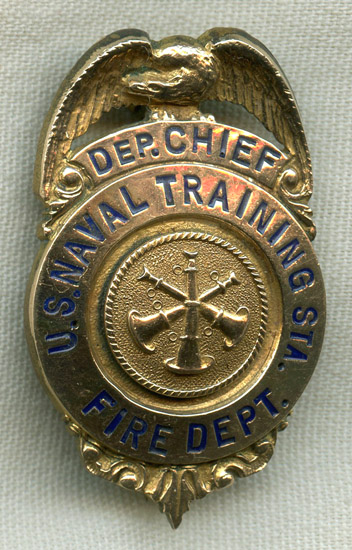The image depicts a gold badge belonging to a Deputy Chief of the U.S. Naval Training Station Fire Department, resting on a white fabric background. At the top of the badge, there is a prominent eagle with wings swooping downward, perched sternly. The badge is intricately detailed, featuring a banner at the top that reads "DEP. Chief," with "U.S. Naval Training STA." inscribed in a circular section below. The bottom of the badge declares "Fire Department" and includes an ornate, almost floral scroll detail. At the center of the badge, there are three crossed bugles, symbolizing the fire service rank. The lettering on the badge is blue, providing a striking contrast to the gold base.